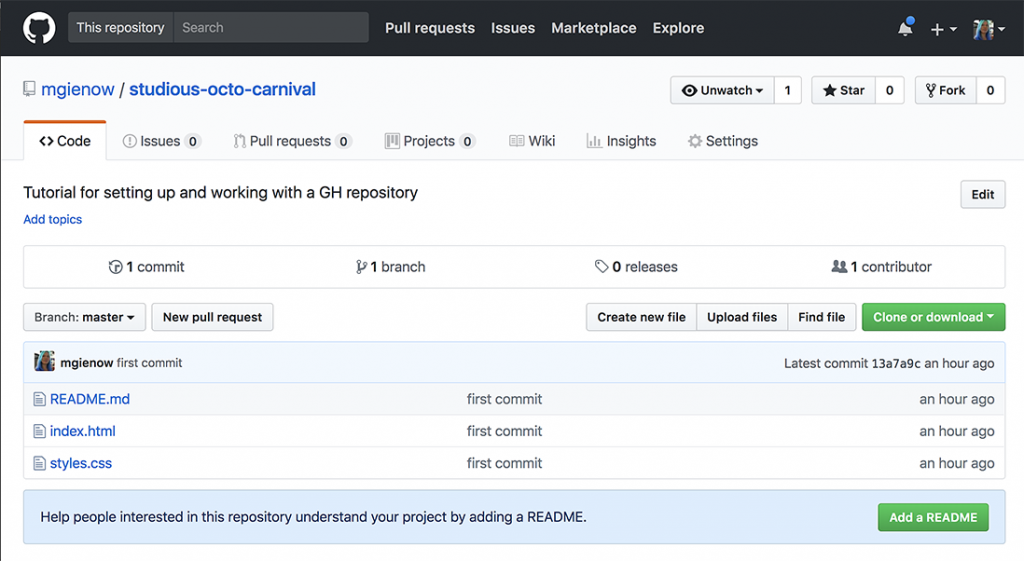This image captures a screenshot of a GitHub repository at the top of the webpage. The repository is named "MGIENOW/studious-octo-carnival." The navigation bar at the top offers various sections including "Pull requests," "Issues," "Marketplace," and "Explore." Below this, additional sections are labeled "Code," "Issues," "Pull requests," "Projects," "Wiki," "Insights," and "Settings."

In the main content area, a heading reads "Tutorial for Setting Up and Working with a GH Repository." Information detailing the repository status includes "1 commit," "1 branch," "0 releases," and "1 contributor." Several links appear at the bottom in blue: "README.md - first commit - an hour ago," "index.html - first commit - an hour ago," and "styles.css - first commit - an hour ago." In the bottom right-hand corner, there is an option to "Add a README."